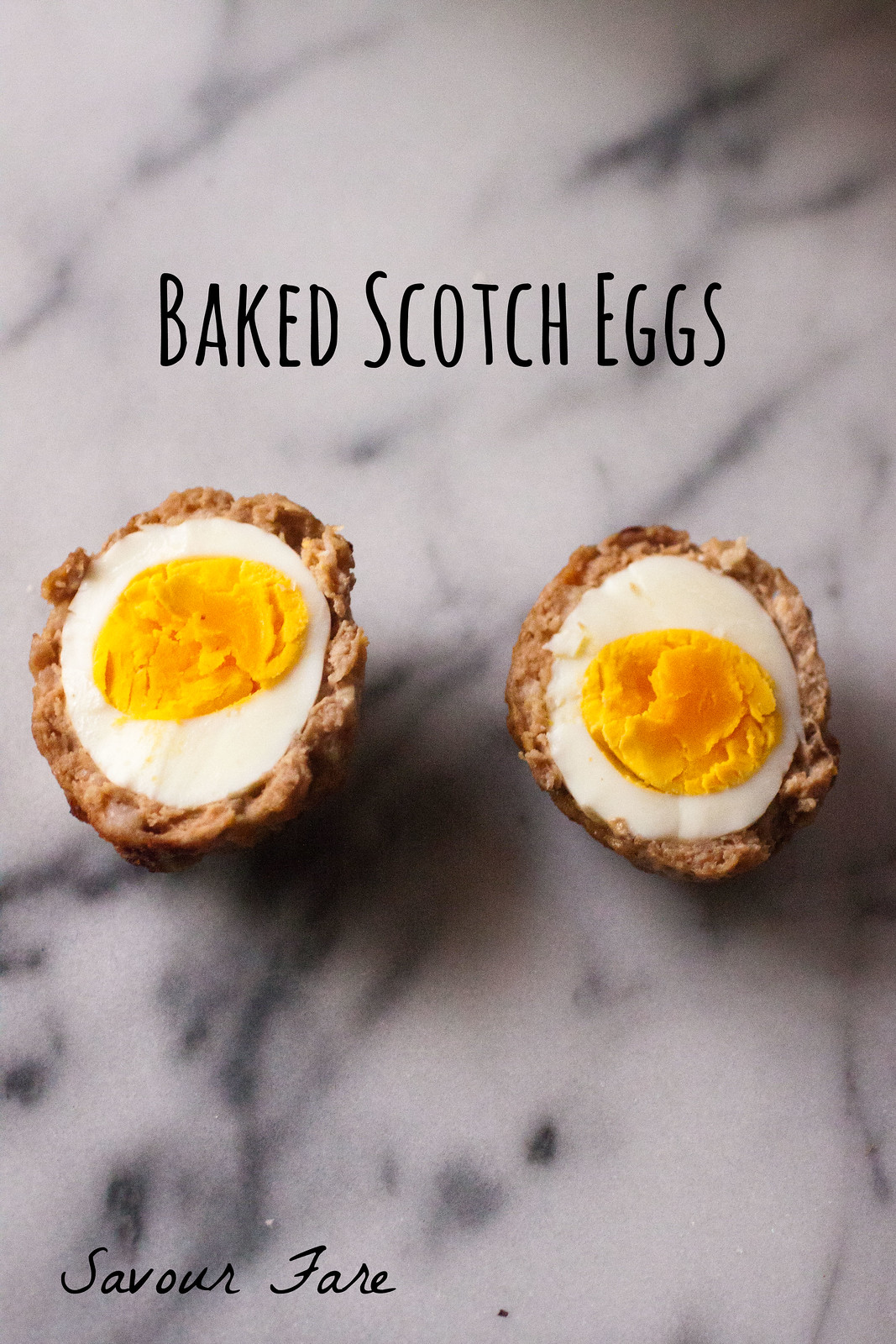The image showcases a pair of baked Scotch eggs, prominently displayed in the center against a subtly blurred white marble or stone countertop, creating an impression of either a kitchen or a restaurant setting. Each egg is meticulously sliced in half, revealing a fully cooked yolk encased in a white, with a brown, crunchy breadcrumb coating enveloping the entire egg. Above these appetizing eggs, the text "Baked Scotch Eggs" is boldly written in black, while in the bottom left corner, additional black text reads "Savoir Faire," potentially indicating the creator or photographer. The colors in the image include shades of off-white, black, white, yellow, brown, and gray, contributing to a visually appealing presentation that hints at a sophisticated culinary advertisement.